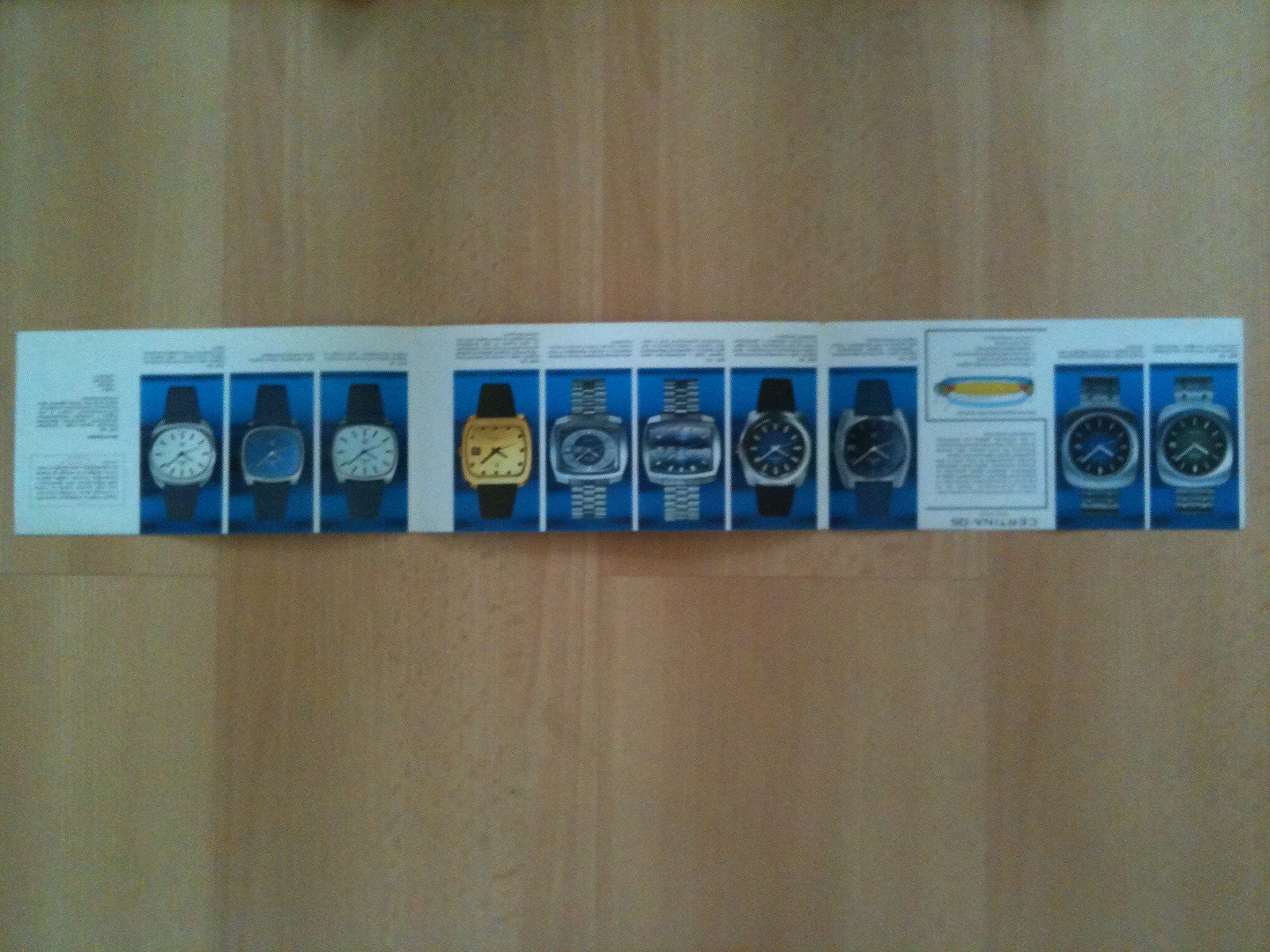This photograph captures a long rectangular piece of white paper promoting a variety of wristwatches, displayed on a light brown wooden surface. The paper, reminiscent of an advertisement or literature from a watch dealer, features an array of wristwatches organized in a single row against a blue background. On the left side, three watches are positioned side-by-side: the first with a white face, the middle one with a blue face, and the third with a white face, all adorned with distinct black armbands. Moving to the center, there are five watches: the first with a gold face and brown band, followed by two silver watches with matching silver faces and bands, then two watches with black faces and silver borders on black bands. The end of the row showcases two more watches with black faces, silver frames, and silver bands. The tiny black text on the paper is illegible from this angle, and the entire layout, including both the text and images, appears inverted, suggesting the photo was taken from an overhead view looking down at the upside-down display.